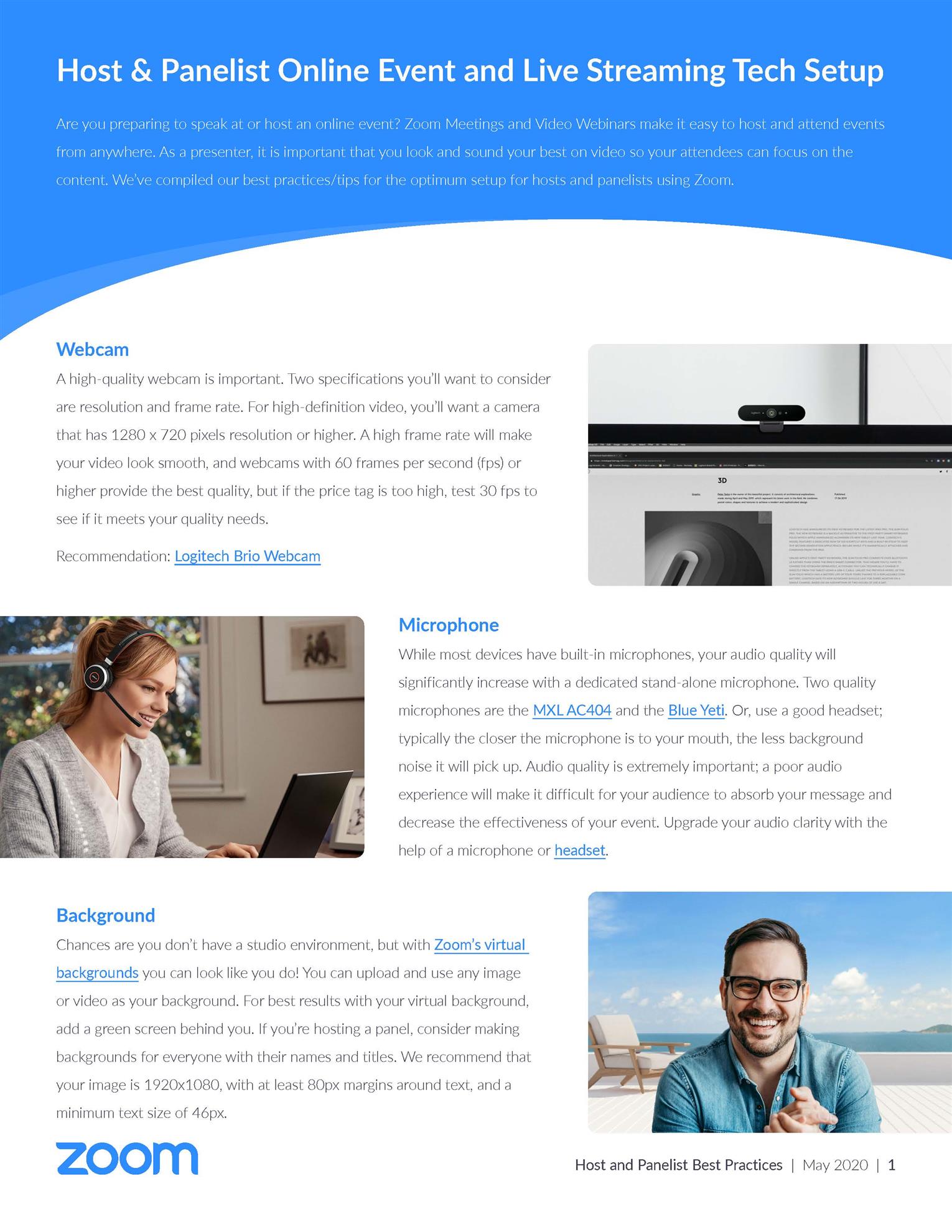Here is a detailed and cleaned-up caption for the descriptive image:

---

**Informational Page on Preparing for Online Events with Zoom**

The webpage features a white background, except for the top section, where a blue concave curve and a blue banner embellish the header. White text is displayed prominently within this blue area.

**Header:**
- *Large Title:* "Host and Panelist Online Event and Live Streaming Text Setup."
- *Subheader Paragraph:* "Are you preparing to speak at or host an online event? Zoom meetings and video webinars make it easy to host and attend events from anywhere. As a presenter, it is important that you look and sound your best on video so your attendees can focus on the content. We've compiled our best practices tips for the optimum setup for hosts and panelists using Zoom."

**Content Section:**
Beneath the blue header, the white section of the webpage is organized into several informative paragraphs, each with a blue title.

1. **Webcam:**
   - *Paragraph:* "A high-quality webcam is important. You'll want to consider resolution and frame rate. For high-definition video, you'll want a camera that has 1280 by 720 pixels resolution or higher. A high frame rate will make your video look smooth, and webcams with 60 frames per second (FPS) or higher provide the best quality. But if the price tag is too high, test 30 FPS to see if it meets your quality needs."
   - *Recommendation (in gray text):* "Logitech Brio webcam" (presented in blue underlined text).
   - *Visual Accompaniment:* An image of a webcam mounted on top of a computer is placed to the right of the webcam paragraph.

2. **Microphone:**
   - *Paragraph:* (To the right of the accompanying image) "Ensure your voice is clear and easy to understand by using a high-quality microphone."
   - *Visual Accompaniment:* A picture of a woman wearing a headset with a microphone.

3. **Background:**
   - *Paragraph:* (To the right of the accompanying image) "Choose a background that is professional and free of distractions. A virtual background can also be a good option, such as an office setting or a serene outdoor scene."
   - *Visual Accompaniment:* An image showing a man sitting in front of a fake ocean view.

The layout is designed for easy reading, providing valuable information and visual aids to help hosts and panelists optimize their setup for Zoom events.

---